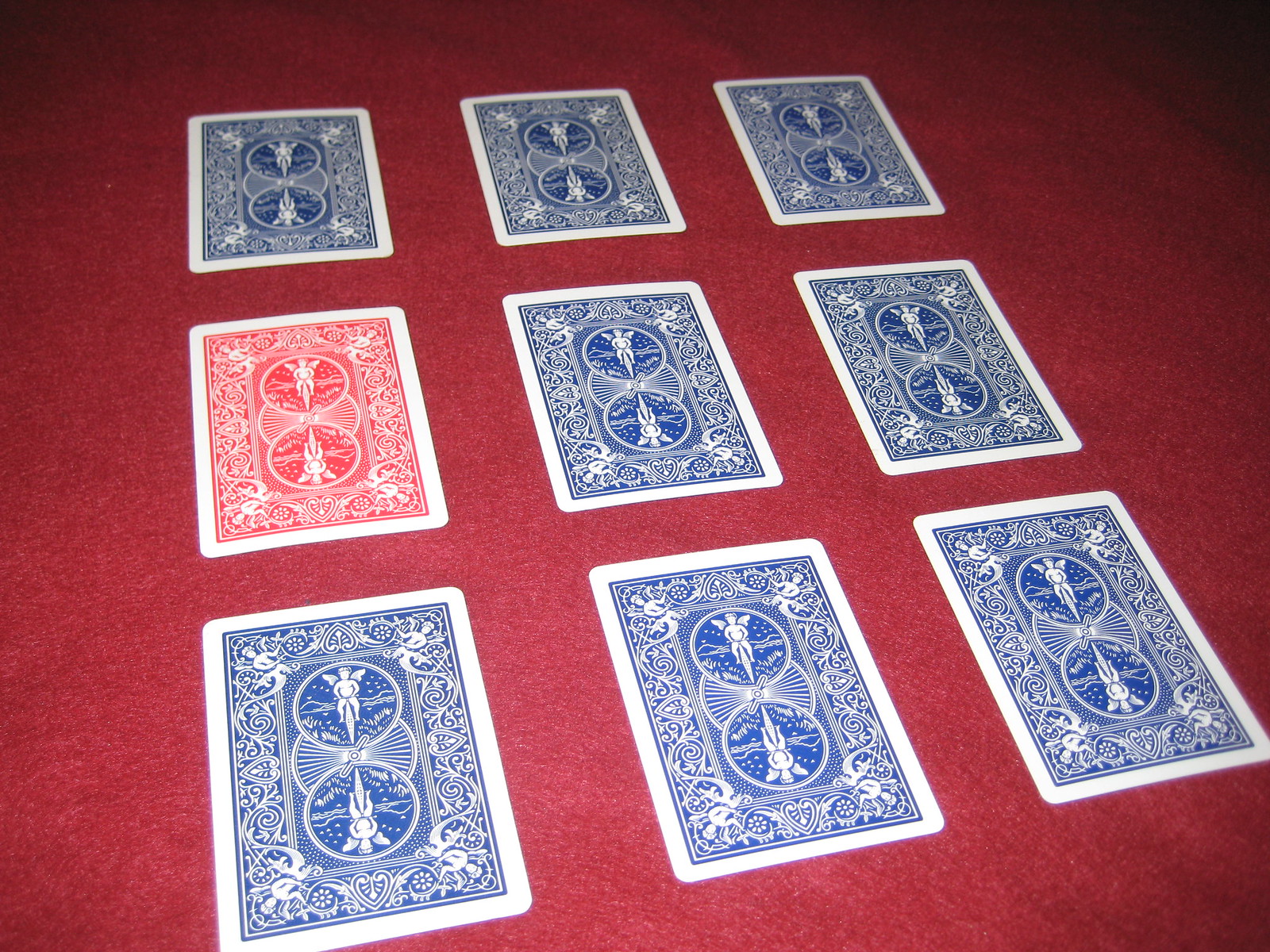The image depicts nine playing cards arranged against a vibrant red background. The cards occupy approximately three-fourths of the image, leaving narrow borders of red on the left and right sides—about an eighth of the width on the left and a tenth on the right. There is no red background visible at the top, and only a small margin is present at the bottom.

In a grid formation, the cards are organized into three rows, with three cards in each row. The top row consists entirely of blue cards. In the middle row, the leftmost card is red, followed by two blue cards. The bottom row is made up entirely of blue cards.

Each card features an intricate design that includes images of cherub angels. Specifically, the design showcases two central cherub angels surrounded by four additional angels. This motif is consistent across all nine cards, including the solitary red card.